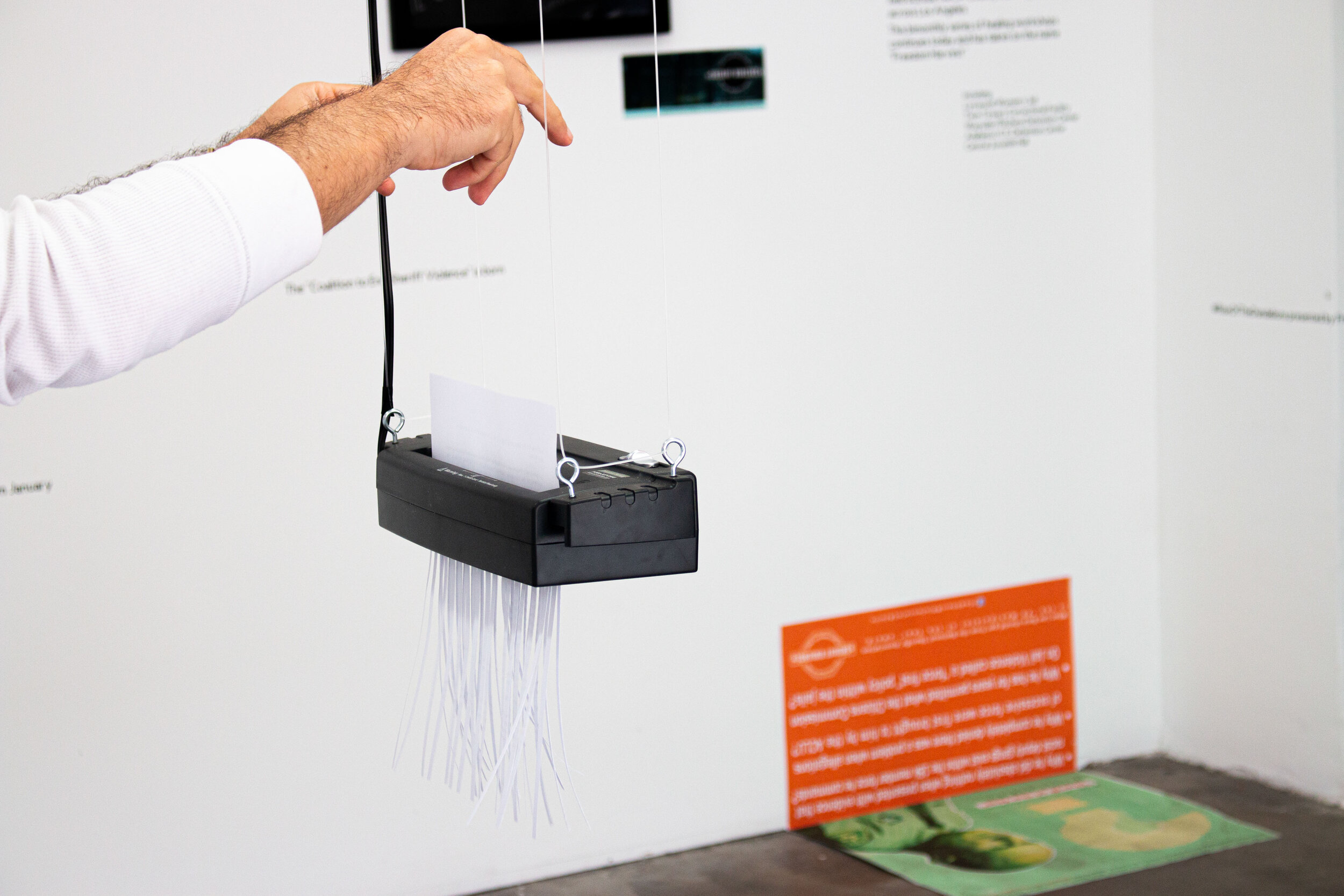The image depicts a corner of a room with white walls and a dark brown floor, resembling a real-life photograph of an art or science demonstration. The walls have various areas of black text, including quotes and a couple of black rectangular shapes near the top. In the center of the back wall, a black paper shredder is suspended from the ceiling by white strings. A pair of men's hands, wearing a long-sleeved white shirt, are feeding a piece of paper into the shredder, with shredded paper dangling below. On the floor in the bottom right corner, there is an orange sign with text propped up against the wall, and a green sign featuring a question mark and the image of a man lying down.